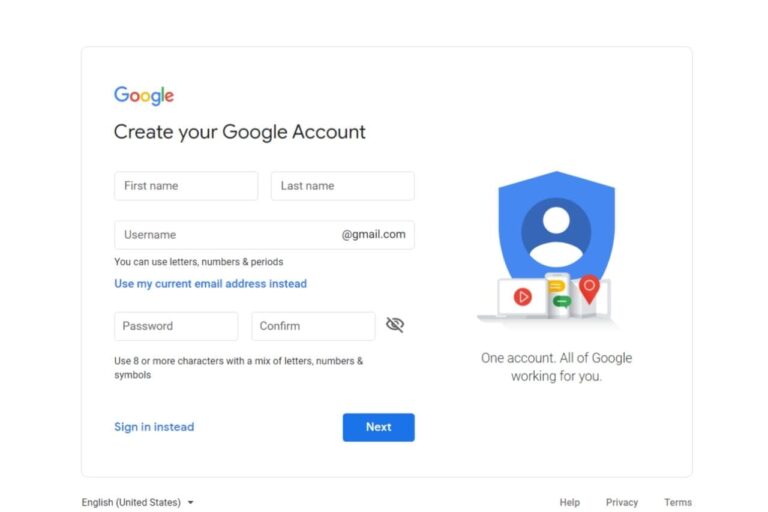This is a screenshot of the Google Account creation page. At the top left corner, there's the familiar Google logo composed of a blue 'G', red 'O', yellow 'O', blue lowercase 'g', green 'L', and red lowercase 'e'. Below the logo, a bold black title reads "Create your Google Account". Immediately underneath, there are text fields for entering your first name, last name, and a username that's appended with "@gmail.com". A note below the username field advises that you can use letters, numbers, and periods. There's also a blue hyperlink reading "Use my current email address instead" for those who prefer to sign up with a non-Gmail address. Following these fields, there are additional fields for setting and confirming a password, accompanied by an ey icon that is crossed out, suggesting a feature to view the password. To the right side of the form, there is a blue shield icon featuring an avatar, with a caption beneath it that reads "One account. All of Google working for you."